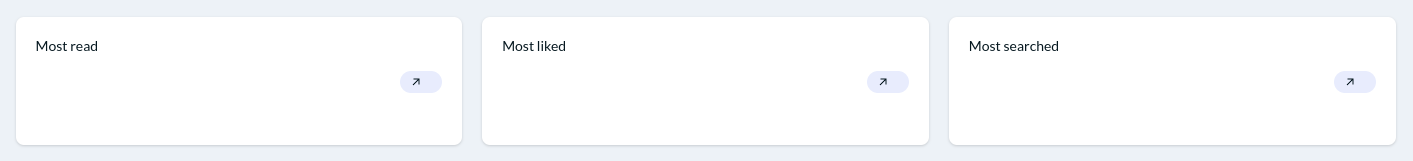A close-up view of a webpage section, prominently featuring three content categorization boxes on a background with a light grayish-blue hue. Each box is distinctively labeled in the upper left-hand corner in black text. 

The first box, situated in the upper left corner, reads "MOST READ" (with "MOST" in capital letters and "READ" also in uppercase). Adjacent to this label, an oval matching the background color contains an arrow pointing diagonally to the right.

The second box, just below the first, is similarly styled and labeled "MOST LIKED" (with "MOST" in uppercase letters and "LIKED" fully capitalized). It also features a corresponding oval with a rightward-pointing arrow.

The third and final box beneath the previous two is tagged "MOST SEARCHED" (with "MOST" in capitals and "SEARCHED" fully uppercase). It includes an oval akin to the others, with the same diagonal arrow pointing to the right.

Each of these boxes seems to offer quick navigation or highlights related to "Most Read," "Most Liked," and "Most Searched" content, providing a streamlined and user-friendly interface.